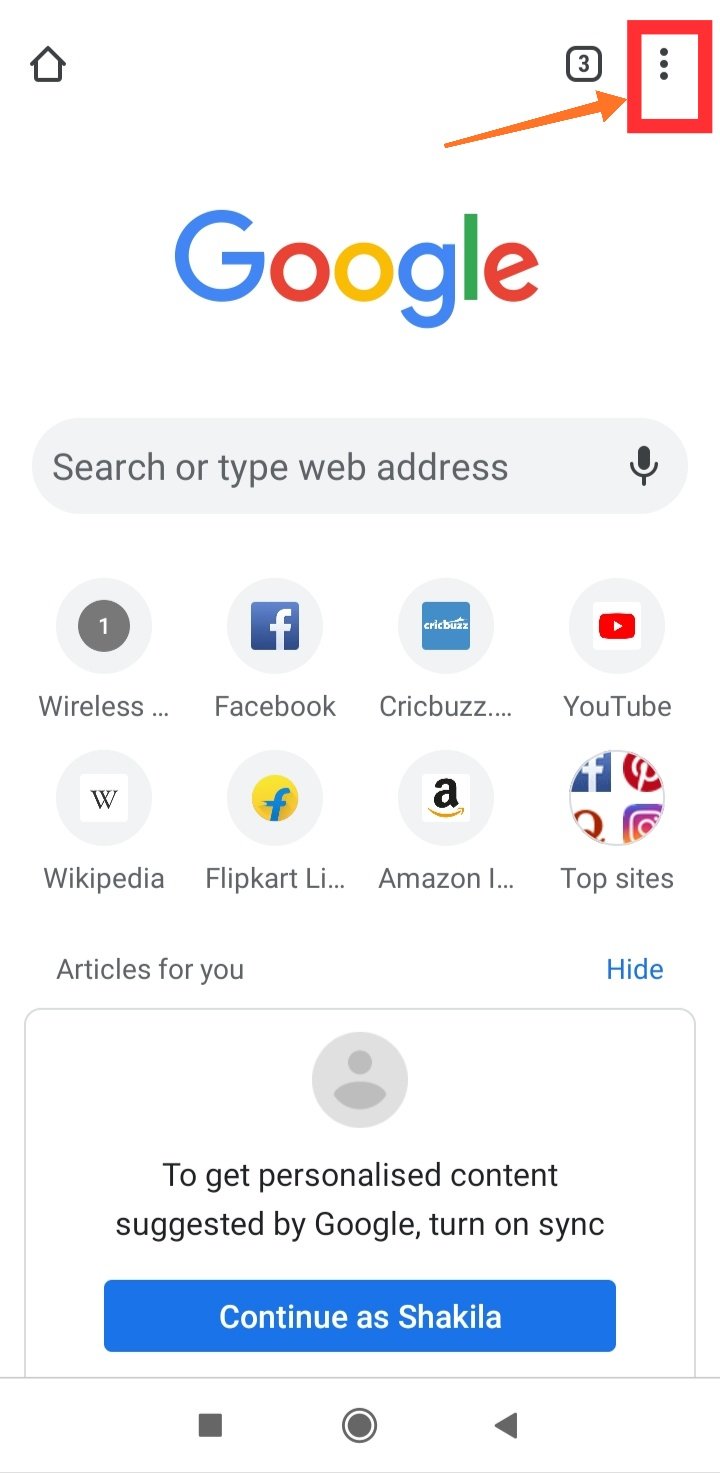The image appears to be a screenshot taken on a smartphone, showcasing a web browser interface. In the upper left-hand corner, there is a small black icon resembling a house, likely representing the home button. On the upper right-hand side, there is a square with the number "3" inside it, and next to it, three vertical dots indicating a menu. 

Highlighted in red with an orange arrow pointing to it, this menu draws attention. At the center of the screen, the word "Google" is prominently displayed with each letter in different colors: the capital "G" in blue, the first "o" in red, the second "o" in yellow, the "g" in blue, the "l" in green, and the "e" in red. Below this, there is a search bar with the placeholder text "Search or type web address," accompanied by a microphone icon for voice search.

Displayed underneath the search bar are several app icons in a grid format:
1. A circle labeled "1," indicating "Wireless."
2. A blue square with a white "F," labeled "Facebook."
3. Another blue square labeled "CricBuzz."
4. A red rectangle with a white play triangle, labeled "YouTube."
5. A circle with a "W," labeled "Wikipedia."
6. A yellow circle with a green "F," labeled "Flipkart."
7. A square with an "A," labeled "Amazon."
8. A circle with the letters "FP" and the Instagram icon, labeled "Top Sites."

At the bottom of the display, a rectangular banner prompts the user to "Get personalized content suggested by Google, turn on sync," with a blue button inviting the user to "Continue as Shaquilla."

Overall, the screenshot captures a comprehensive view of a personalized web browser home screen, featuring quick access to popular websites and services.